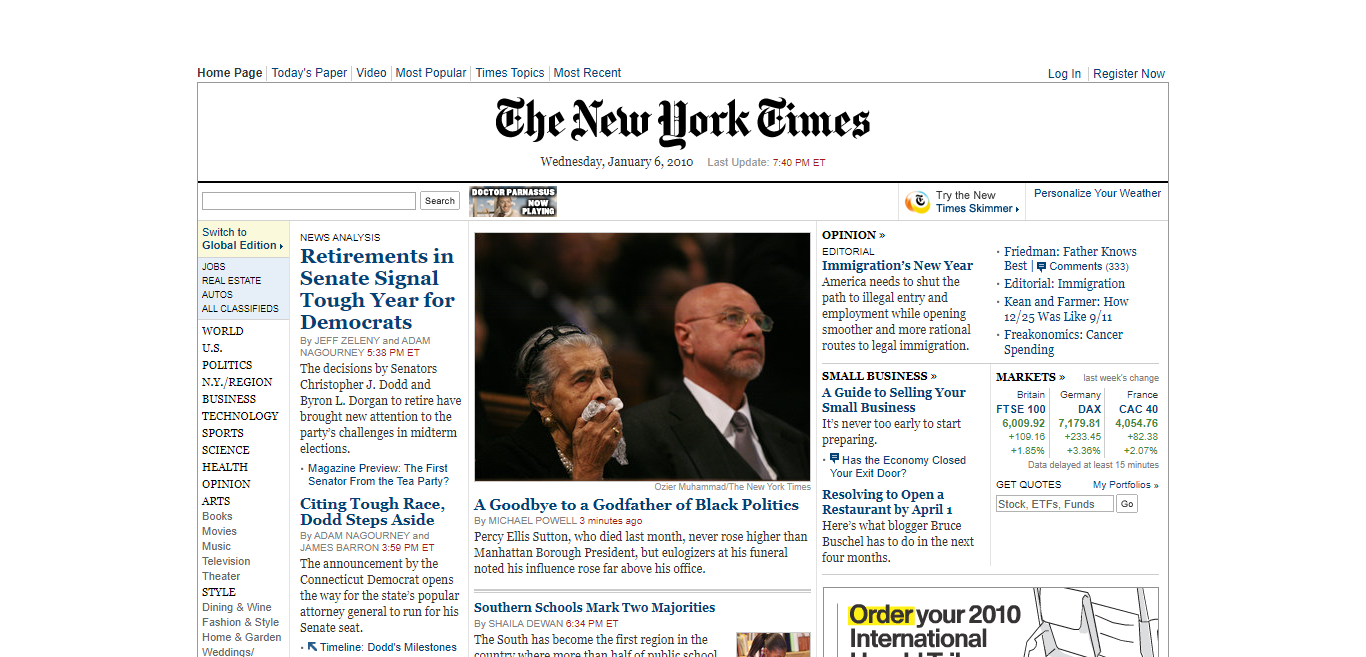This is a detailed description of the New York Times web page as observed on January 6, 2010. 

The background of the page is white. Starting from the top left corner, moving left to right, the navigation bar displays: "Home Page," "Today's Paper," "Video," "Most Popular," "Times Topics," and "Most Recent." On the top-right corner, there are options to "Log In" and "Register Now." 

Centered at the top of the page is the iconic "New York Times" logo. Below, the date "Wednesday, January 6, 2010" is displayed, and it notes the page was last updated at 7:40 PM ET.

Along the left-hand side is an extensive menu of links including categories such as "World," "U.S. Politics," "New York Region," "Musings," "Techno," "Sports," "Science," "Health," "Opinion," and "Arts," followed by smaller links that are difficult to read.

Headlines dominate the main body of the page. The first headline reads: "Retirements in Senate Signaled Tough Year for Democrats," with a sub-headline below stating: "Citing Tough Race, Dodd Steps Aside." 

In the middle section is a picture of two individuals, one holding a handkerchief to their mouth. The caption beneath the image reads: "A Goodbye to Godfather of Black Politics."

On the right-hand side are further sections including "Opinion," "Editorial," "Small Business," and at the bottom right, there's an advertisement with the text: "Order your 2010 International."